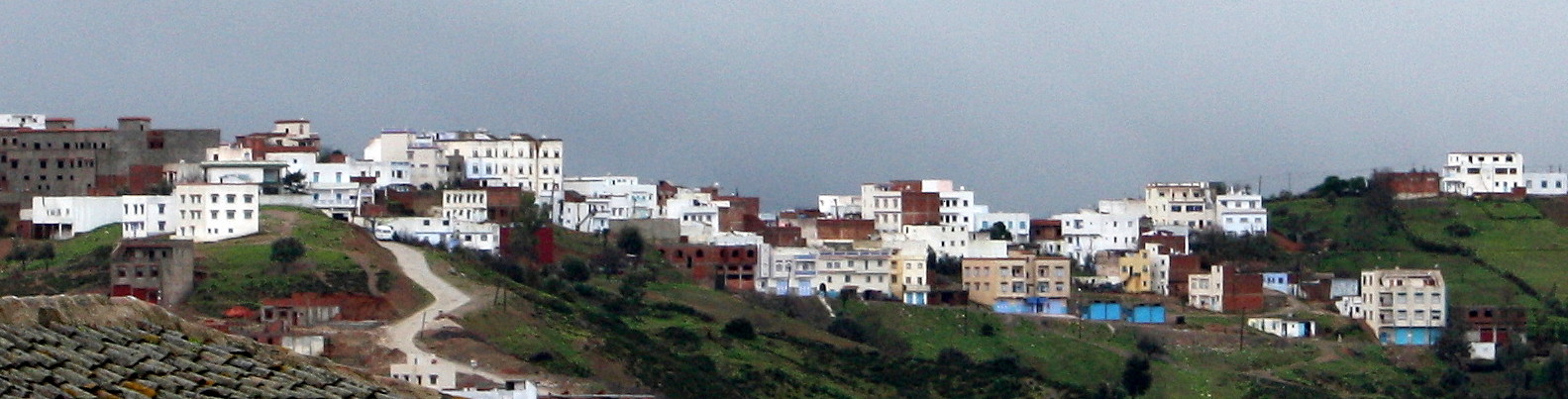The image portrays a panoramic view of a sprawling hillside town, depicted in a rectangular, elongated photograph. The scene captures a vast expanse of the area, emphasizing its wide, left-to-right orientation. A significant portion of the town's architecture consists of numerous, closely-packed white and tan buildings, many of which exhibit multiple windows indicative of apartment-style housing. Nestled among these structures are a few brown buildings, adding some color variation to the predominantly pale landscape.

The hillside itself is dotted with greenery, consisting of grassy patches, bushes, and scattered trees, which collectively add a lush contrast to the stone and concrete facades of the buildings. A dirt or gravel road can be observed meandering down the left side of the hill, providing access to the homes and connecting them to the rest of the landscape. In the bottom left-hand corner, a tiled roof suggests the viewpoint is from another building situated on the hill.

The sky overhead is a brilliant, uninterrupted blue, free from any clouds, enhancing the clarity and brightness of the scene. This broad, panoramic shot encapsulates the serene yet expansive nature of the hillside town, offering a comprehensive glimpse of its architectural layout and surrounding natural beauty.